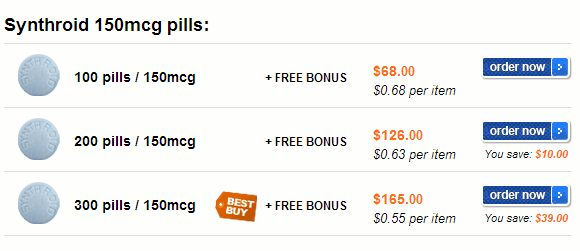The image shows a digital page with detailed information about purchasing Synthroid, a medication used for thyroid hormone replacement. At the top of the page, the name "Synthroid," spelled S-Y-N-T-H-R-O-I-D, is prominently displayed alongside a description of the dosage, which is 150 MCG (micrograms) per pill.

Below the title, there are three sections, each featuring an image of a pill and specifying different quantities available for purchase. The first section offers 100 pills at 150 MCG each, priced at $68, equating to $0.68 per pill. The second section lists 200 pills at the same dosage for $126, making each pill $0.63. The third section, highlighted with an orange tag that reads "Best Buy," provides 300 pills for $165, bringing the cost down to $0.55 per pill.

Each section also includes a note stating "+ Free Bonus" in black print. At the bottom of every section, a blue "Order Now" button is prominently displayed, inviting users to make a purchase.

This meticulously organized page provides a clear comparison of the different purchasing options, highlighting the most cost-effective choice, and encouraging quick purchasing decisions.